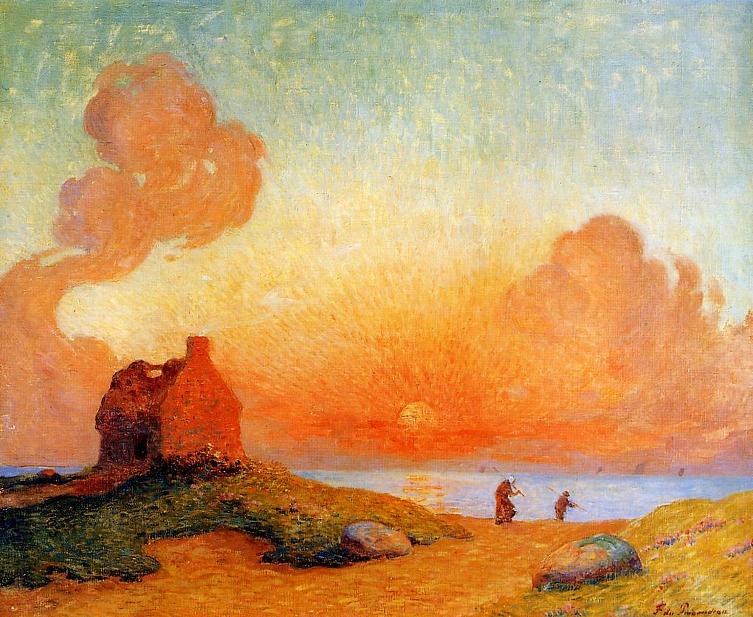This image, painted in a style reminiscent of Van Gogh, vividly captures a fiery sunset or sunrise. The sky dominates the scene with intense shades of orange and yellow, transitioning to splotches of blue, light green, and white near the top. The sun appears as a radiant yellow semicircle on the horizon, which sits about one quarter up from the bottom edge of the painting. Radiating from the central sun are vibrant orange clouds that swirl across the sky, suggesting a dynamic and almost stormy atmosphere.

Below the horizon, a light blue body of water mirrors the sun’s colors. The water is bordered by a sandy shore, depicted in rich orange hues, while the bottom right corner features a golden tone. On the left side of the shore, a green mossy patch supports an orange structure resembling a small house or old brick building, with a little chimney, possibly abandoned given its dilapidated top. In the lower right, two small figures are visible, carrying sticks over their shoulders as they approach the water. These figures, clad in garments with red and brown tones, add a narrative element to the tranquil yet fiery landscape. Boats can be faintly seen on the horizon, adding to the scene’s depth and story.